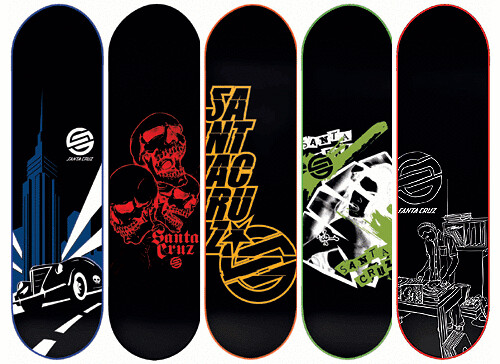This image features five black skateboards laid out side-by-side in a top-down perspective, each showcasing unique and vibrant artwork. The first skateboard depicts a blue Empire State Building with white spotlights streaming from its base, accompanied by a vintage black automobile with white rims driving on a black road. A partially visible logo is also present near the skyscraper. The second skateboard displays three red skulls outlined in black, with "Santa Cruz" written beneath them in bold red letters. The third skateboard features the "Santa Cruz" name split across multiple lines in bright yellow letters, arranged in a vertical column, with a star and a complex circular logo at the top. The fourth skateboard has an intricate illustration resembling playing cards with a green ooze splatter in the background and the "Santa Cruz" logo subtly incorporated into the design. The fifth and final skateboard showcases a white outline drawing of a giant man climbing what appears to be the Empire State Building again, set against the black background, making the design striking and prominent. The detailed illustrations on each skateboard stand out vividly against their dark backgrounds, creating a captivating visual array.